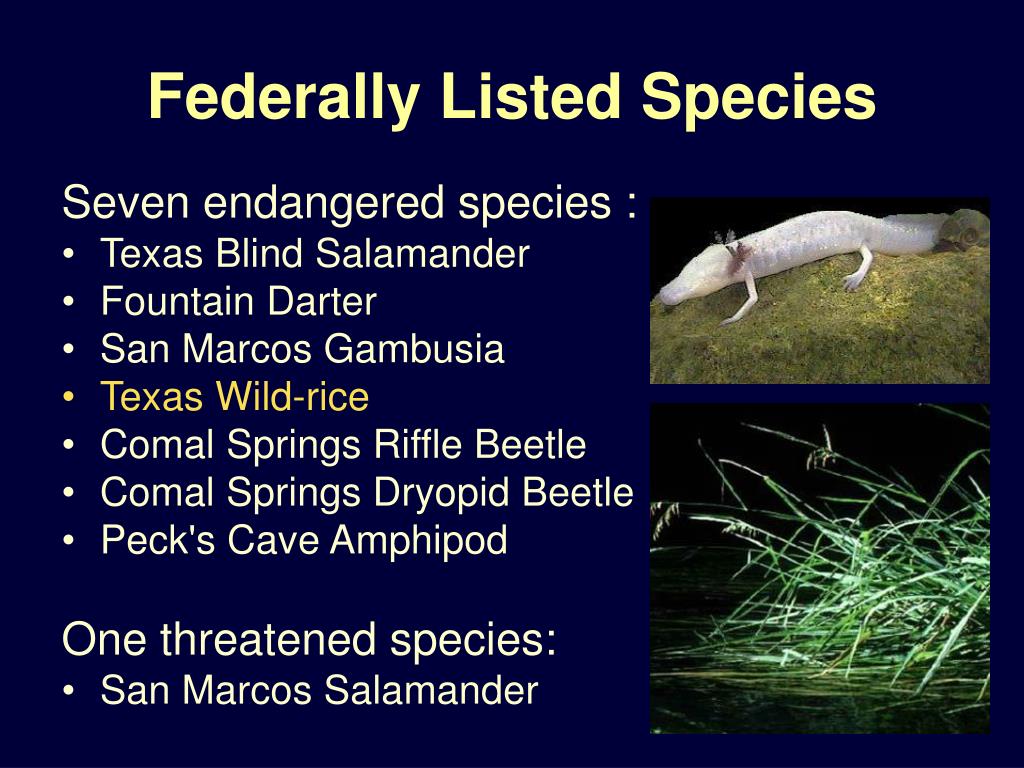The image is a detailed PowerPoint slide with a dark blue background that prominently features the title "Federally Listed Species" in bold yellow text, centered at the top. On the left side of the slide, white text outlines a list of species: "Seven Endangered Species," followed by bullet points naming the Texas Blind Salamander, Fountain Darter, San Marcos Gambusia, Texas Wild Rice, Comal Springs Riffle Beetle, Comal Springs Dryopid Beetle, and Pex Cave Amphipod. Below this, it states "One Threatened Species," with the bullet point listing the San Marcos Salamander. To the right of the text, there are two images: the top image shows the Texas Blind Salamander, a creamy-colored, eyeless amphibian with four legs and what appear to be ear-like structures. The bottom image features Texas Wild Rice, depicting green, grass-like leaves emerging from the water.